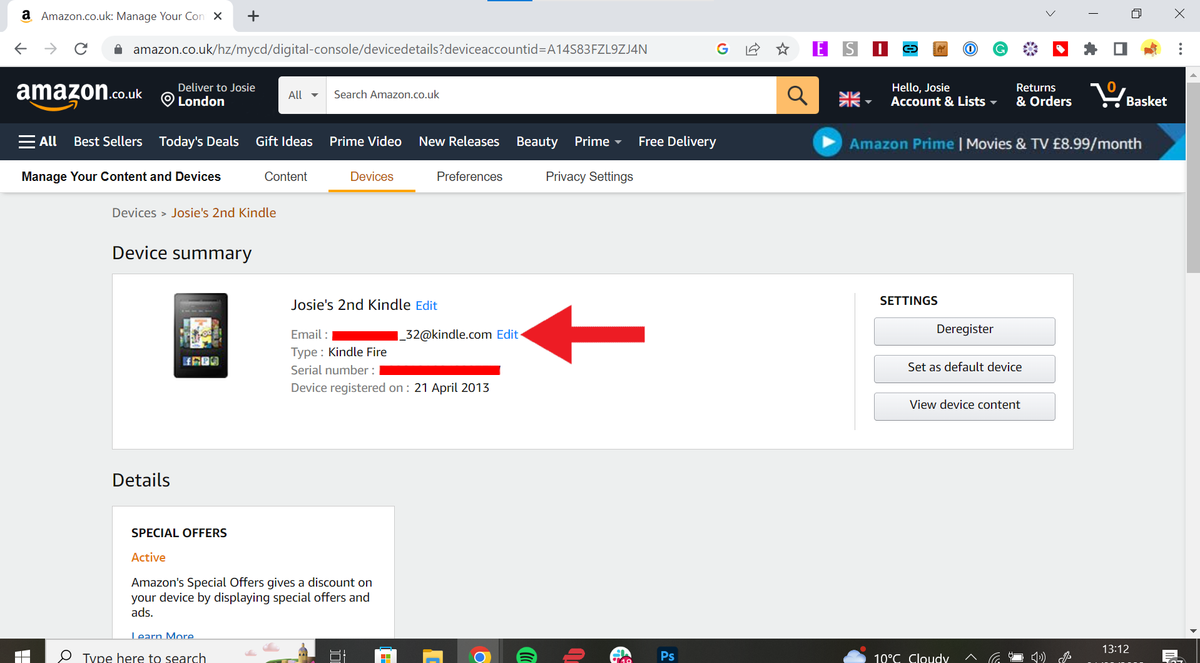**Amazon.co.uk - Manage Your Devices Page for Josie's Second Kindle**

This image is a screenshot of an Amazon web page from the Amazon.co.uk domain, specifically focused on managing devices under the user account named Josie. At the top of the page, the well-known Amazon logo is prominently displayed alongside the partially visible label "Amazon Cloud Manage."

Below the header, a search bar is positioned prominently, allowing users to "search all Amazon UK." To the right of the search bar, the page indicates that deliveries are directed to Josie in London. The navigation bar features a British flag icon, followed by a friendly greeting, "Hello Josie," and links to "Account and Lists." The shopping basket icon shows "0," indicating no items are currently in the basket.

The main section of the page is dedicated to device management, specifically for "Josie's second Kindle." Details include a summarized view of the device's essential information:

- **Device Name:** Josie's second Kindle
- **Device Type:** Kindle Fire
- **Device Email Address:** [Hidden for privacy]
- **Serial Number:** [Serial number details]
- **Registration Date:** 21st of April, 2013

There are several actionable options available, such as the ability to "Deregister," "Set as Default Device," and "View Device Content."

Moreover, the status of "Special Offers" is marked as active, indicating that Amazon special offers, which provide a discount on the device in exchange for displaying ads, are enabled. There's also a link to "Learn more" about these offers.

At the bottom of the screen, a toolbar showcases an array of icons linked to various apps, underscoring the multifunctional capabilities of the device.

Overall, the webpage offers a comprehensive and user-friendly interface for managing Amazon devices, with all relevant information and options clearly presented.